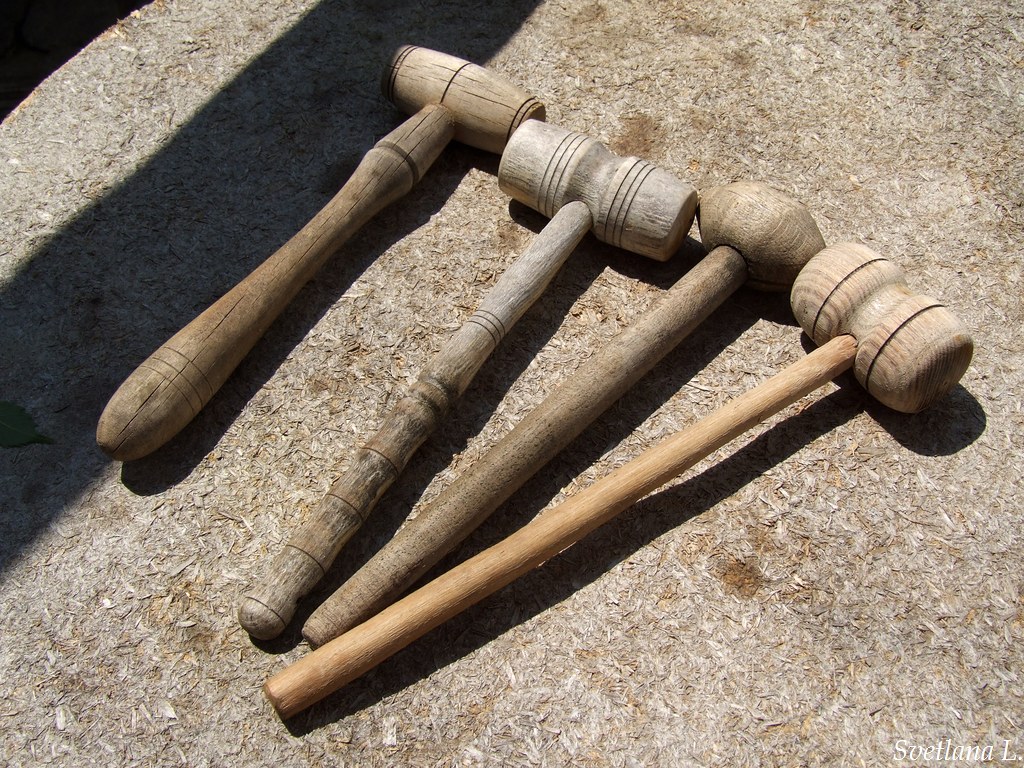The image depicts four distinct wooden mallets with varying designs, laid out on a brown, textured surface that resembles compacted dirt or concrete. The handles of the mallets extend towards the bottom left corner, while their heads point to the top right. Despite their variances, all the mallets share a wooden, predominantly brown composition, ranging from light to darker shades, and some exhibit cracks on their handles. Each mallet casts a defined shadow, suggesting strong sunlight from the top left. 

On the furthest left, the back mallet has a contoured handle and a head shaped like two barrels. Next, the mallet with the slightly textured, bamboo-resembling handle features a cylindrical head with one line in the middle and two lines on the top and bottom. The third mallet, with a thicker handle, boasts an oval-shaped hammering part reminiscent of old-fashioned maces. The frontmost mallet has a slender, longer handle and features two larger cylindrical segments on its hammering head. 

Additionally, there is a green leaf on the left side of the image and the bottom right corner bears white text that reads "Svetlana L." The combination of these elements, along with the shadows and varied lighting, highlights the rustic and well-worn nature of the mallets.